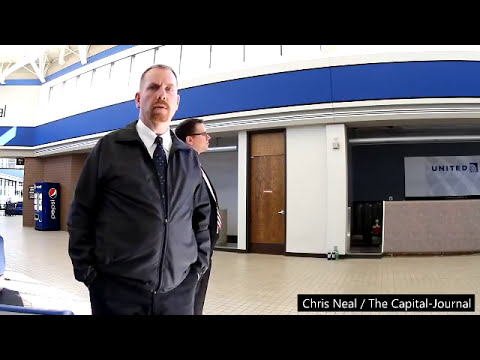The image is a security camera screenshot taken inside an airport, featuring two white male security guards. The main focus is on the first individual, who is facing the camera directly. He appears to be in his 40s, has a receding hairline, short brown hair, and a brown goatee. He is wearing a black zip-up jacket over a white collared shirt, paired with a blue tie adorned with various colored triangles and diamonds. The second individual, positioned slightly behind and to the side, is looking away from the camera. He wears black-framed glasses, a black jacket, and a tie striped in red, white, and blue. The background highlights several key details: a Pepsi vending machine, a brown door, and walls partially made of concrete and brick. Prominently featured is a banner for United Airlines in blue font. The image is credited to Chris Neal of The Capital Journal, with the text placed in the bottom right corner. The overall design of the setting includes blue and white elements, with white tiles on the floor.